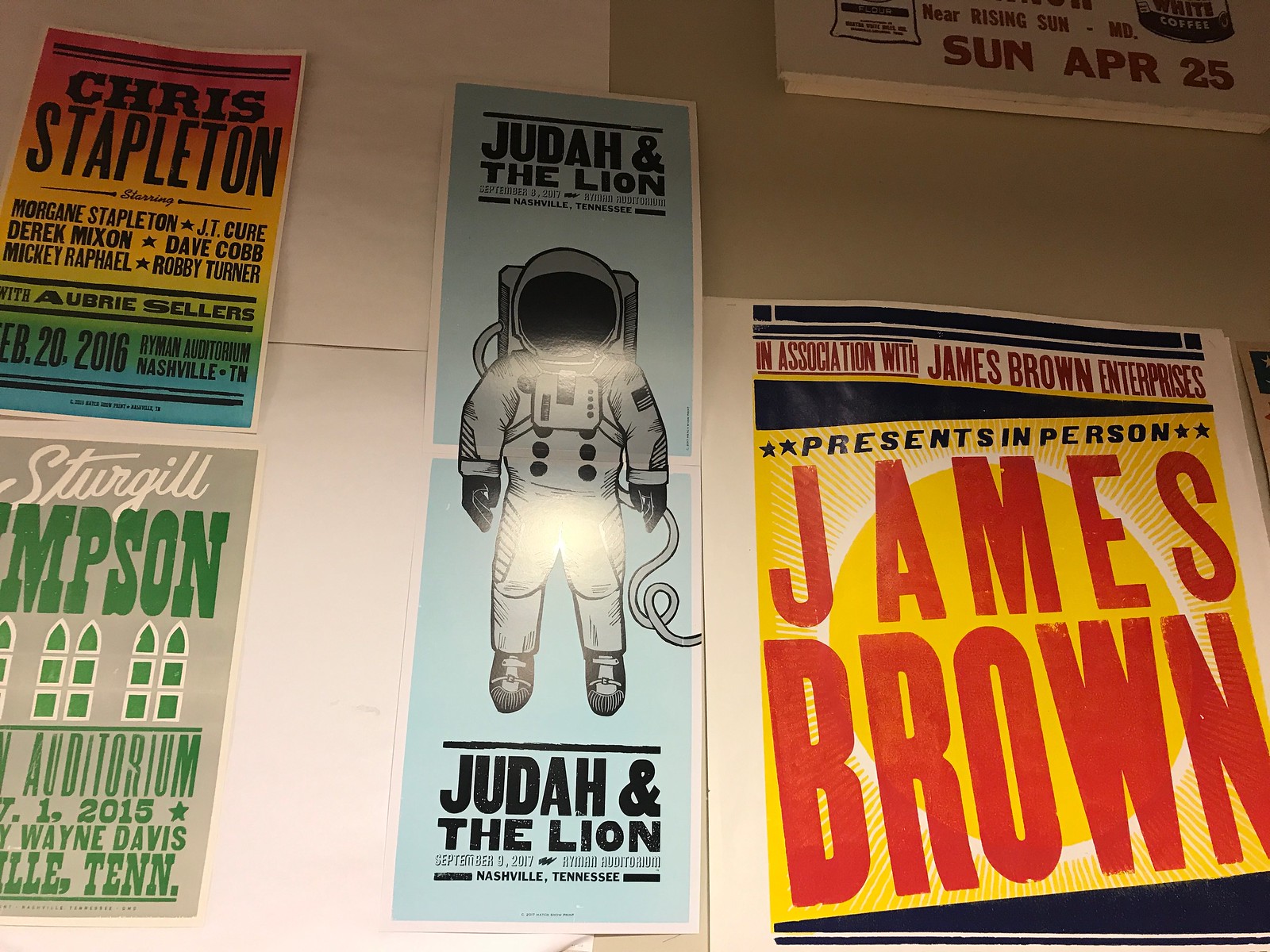In this image, various colorful posters for musical performances are displayed on a wall. The top left features a vibrant poster in red, yellow, orange, green, and blue hues, listing artists like Chris Stapleton, Morgan Stapleton, J.T. Cure, Derek Mixon, Dave Cobb, Mickey Raphael, and Robbie Turner, with Aubrey Sellers, resembling a concert announcement. To the bottom left, a gray poster with green and white lettering partially reads "Sturgill Simpson" and includes the word "auditorium," though it's cut off. Dominating the center is a tall blue poster with an astronaut image, advertising Judah and the Lion, including details about a September performance in Nashville, Tennessee. On the bottom right, a big sign with red letters against a yellow background announces "James Brown Presents In Person," affiliated with James Brown Enterprises. Another poster, partly visible at the top right, features text in red letters on a white background mentioning "Near Rising Sun" and "April 25". The posters are spread out across the wall, creating a vibrant and eclectic display of music-related advertisements.